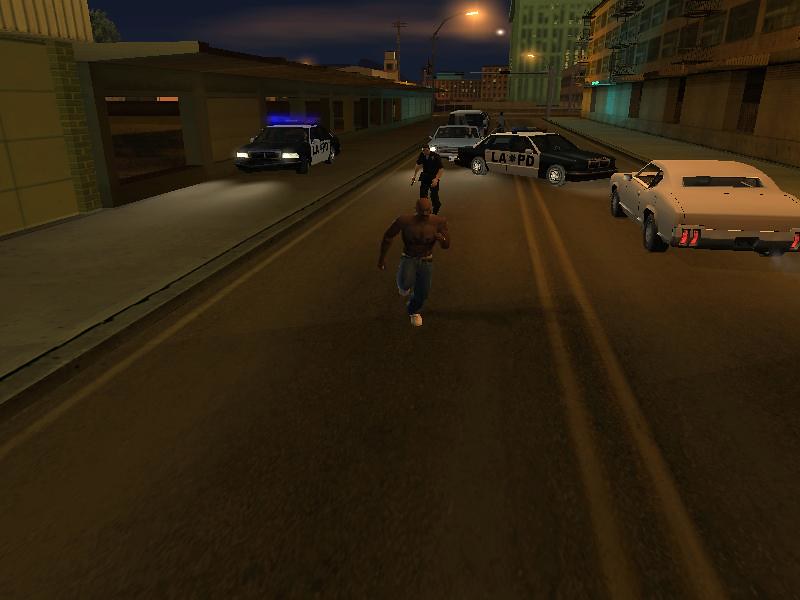The image appears to be a screenshot from an early PlayStation-era video game, characterized by its primitive 3D graphics. The central figure is a shirtless black man wearing blue jeans and white sneakers, captured mid-stride as he runs away from a police officer. The officer, gun drawn, is approximately 15 feet behind him in hot pursuit. The backdrop includes two police cars, one parked on the curb and the other stationed in the middle of the street, both prominently marked with "LAPD" on their sides.